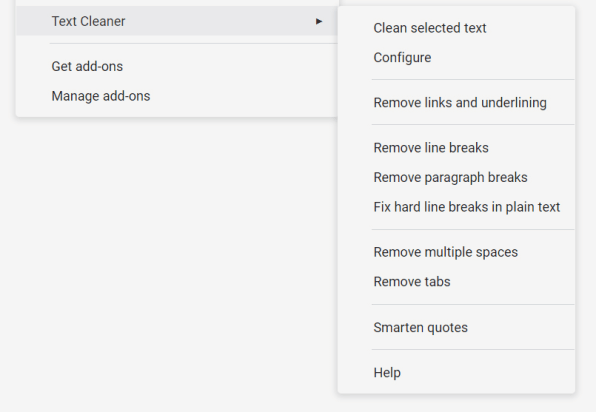In this image with a light gray background, the layout is divided into two sections. On the left side of the image, there are three text elements stacked vertically: 

1. "Text Cleaner" positioned at the top left corner.
2. "Get Add-ons" located directly below "Text Cleaner."
3. "Manage Add-ons" found directly below "Get Add-ons."

The right side of the image features content within the "Text Cleaner" tab, presenting a series of options in a vertical list from top to bottom. These options include:

1. "Clean Selected Text"
2. "Configure"
3. A very thin horizontal line
4. "Remove Links and Underlining"
5. Another thin horizontal line
6. "Remove Line Breaks"
7. "Remove Paragraph Breaks"
8. "Fix Hardline Breaks in Plain Text"
9. Another thin horizontal line
10. "Remove Multiple Spaces"
11. "Remove Tabs"
12. Another thin horizontal line
13. "Smart in Quotes"
14. Another thin horizontal line
15. "Help"

The image is primarily square-shaped, with a light gray background that encompasses the entire scene.